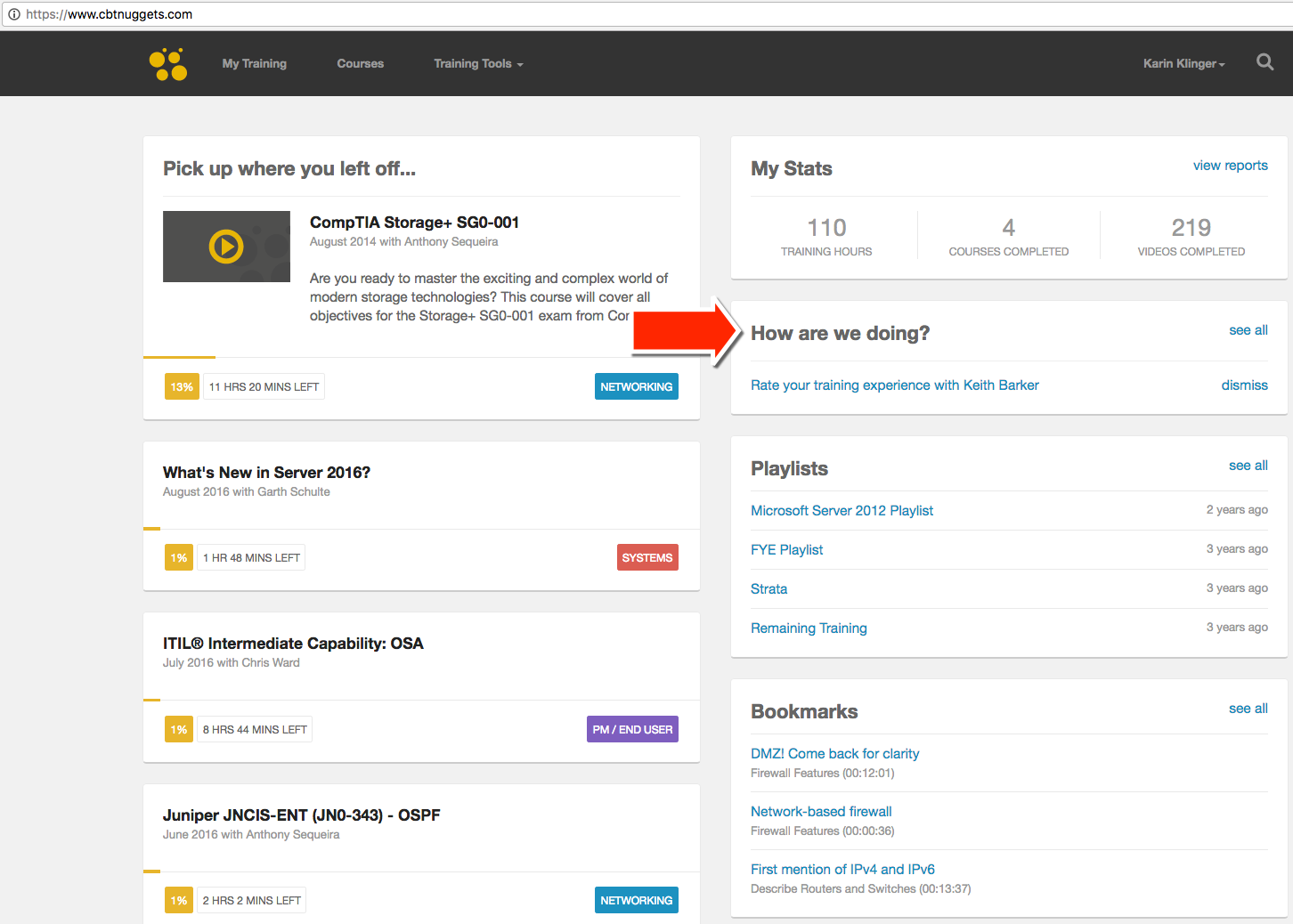The screenshot displays a webpage from CBT Nuggets, visible via the address bar in the upper left corner, which reads "www.cbtnuggets.com." Below this, a black banner spans the width of the page, featuring a geometric logo consisting of four yellow circles and two yellow dots. To the right of the logo are navigation links including "My Training," "Courses," and "Training Tools," each accompanied by a pull-down arrow, and in the upper right corner, "Karen Klinger" with another pull-down arrow and a magnifying glass icon for search functionality.

Beneath this banner is a prominently displayed white box containing bold text that reads, "Pick up where you left off." Below this header, it specifies a course titled "CompTIA Storage+ SGO-001" from August 2014, presented by Anthony Secura. An encouraging message follows, asking, "Are you ready to master the exciting and complex world of modern storage technologies?" To the right of this message, a large, bold red arrow points to the right, likely indicating where users can continue their training or find additional information.